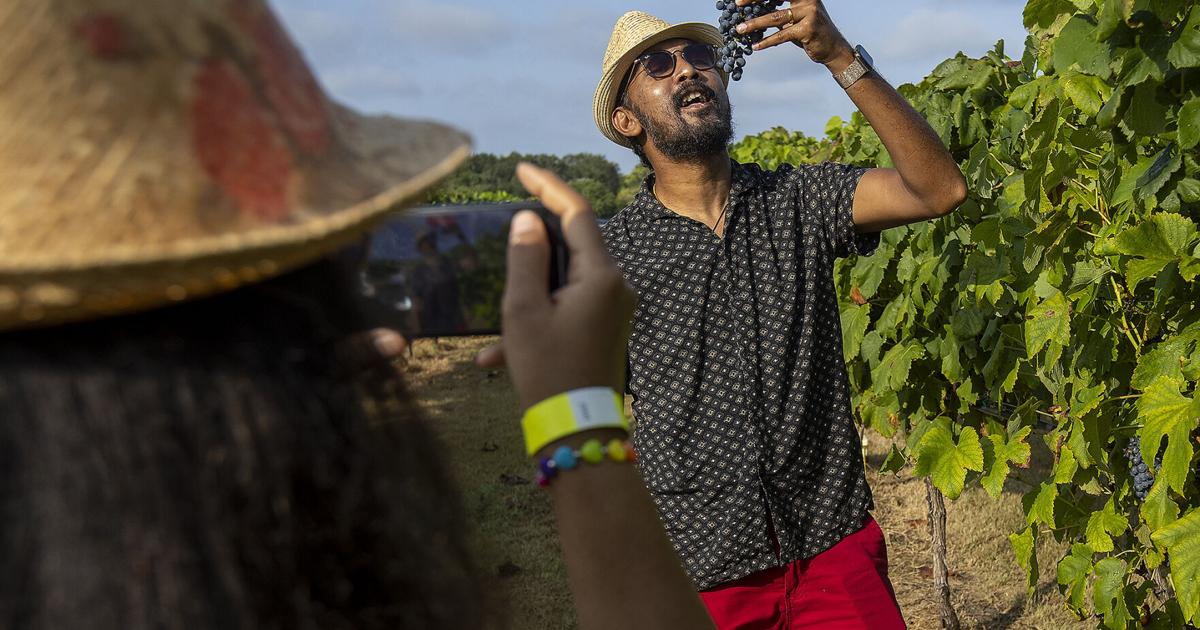In the vibrant setting of a vineyard, a woman with long, dark hair and dark skin stands in the foreground, capturing a moment on her phone. She wears a straw hat and a bracelet with rainbow-colored heart charms. Her subject, a man with dark skin, facial hair, and a scraggly beard, is positioned in the middle ground. He is adorned with a similar straw hat, dark sunglasses, a black t-shirt, red shorts, and a mechanical watch on his wrist. The man is holding a bunch of blue-gray grapes next to his open mouth, posing as though he's about to eat them. Surrounding them, lush grapevines laden with bunches of grapes stretch into the background, set against a sky that is a mix of blue and gray clouds. This picturesque daytime scene is captured from just over the woman's shoulder, adding to the intimate and lively portrayal of a moment in a winery.